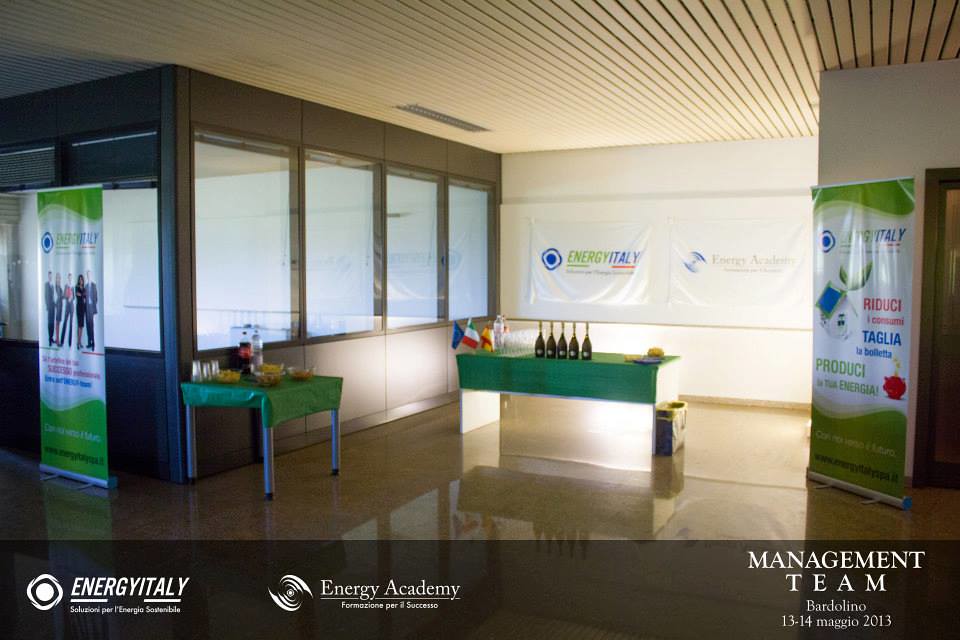The image displays a well-organized reception or workspace area with a polished, shiny terrazzo floor reflecting the surroundings. The ceiling features wood strips, adding to the aesthetic appeal of the room. Central to the scene is a table set up for serving, adorned with five bottles of champagne and small flags. In the background, a white wall prominently displays banners for Energy Italy and Energy Academy, brightly illuminated by a light source.

On either side of the room are promotional banners with green and white backgrounds, each featuring different photographs. The left banner shows people, while the right one has imagery of a house and some small scale or cartoonish graphics along with text. Additionally, a smaller table covered with a green tablecloth holds large bottles of soda and water, bowls of chips, and small plastic cups. The bottom of the image is digitally superimposed with several logos: "Energy Italy," "Energy Academy," and "Management Team, Bartolino, 13-14, Maggio, 2013." The overall setup, including posters and signs about Energy Italy and its products, suggests an event or meeting space, possibly prepared for a reception or a showcase. The room also has multiple windows, adding natural light to the setting.